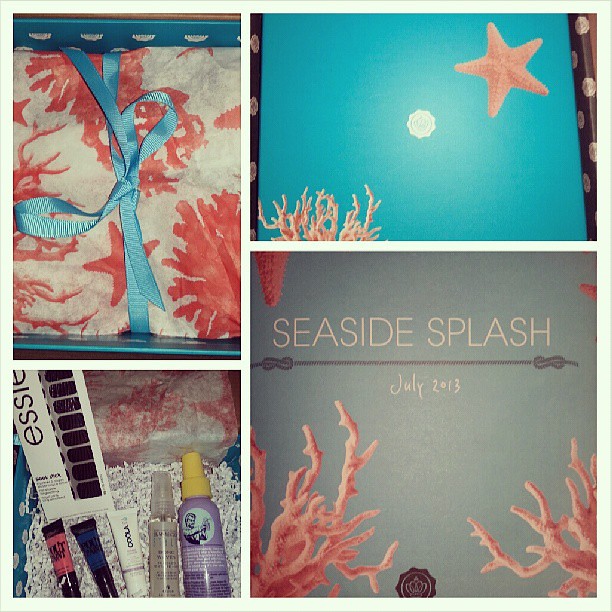The image is a composite photograph divided into four quadrants, each featuring a different seaside-themed subject. 

In the bottom right-hand corner, there is a photograph of a sign that reads "Seaside Splash July 2013" in yellow text against a green background, adorned with a ribbon and bows. The corners of this section also feature red sea coral decorations.

Above this, in the top right quadrant, is an image of a yellow starfish set against a blue backdrop, with additional coral details in the left-hand corner.

The top left quadrant showcases a neatly wrapped package in white and orange, tied with a sea blue ribbon. The package features pink starfish and sea coral designs.

The bottom left quadrant displays an assortment of beauty products, including four tubes and a bottle of hairspray, alongside a box of fake fingernail tips labeled "ESSIE". The box is filled with shredded paper, adding to the texture of the display.

Altogether, the photograph captures a beach-inspired theme with elements of the sea intricately integrated into each quadrant, creating a cohesive and visually engaging collage.